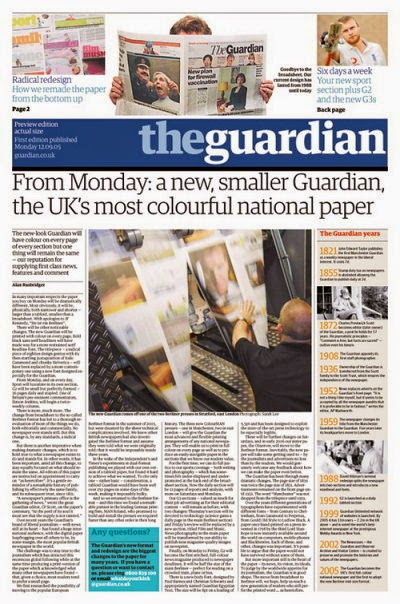This is a detailed screenshot from The Guardian. In the top left corner, there is an image featuring various newspapers with the headline, "Radical Redesign: How We Remade the Paper from the Bottom Up." Central to the image is a person holding up a newspaper, obscuring their face entirely. The back of this newspaper shows a dramatic photograph of a police officer pulling on a man's ears, with the officer positioned just behind the man's left shoulder. The man appears distressed, his mouth open wide. 

On the front cover of the newspaper being held, there is an image of a woman either standing or sitting at a desk in what seems like an office environment. She is dressed in a formal suit, and there is a lamp positioned behind her. 

In the top right corner of the screenshot, text reads, "Six days a week, your newspaper section plus G2 and G3." Below this is a blue header with the title "The Guardian." Beneath the header, against a white background with black text, it announces, "From Monday, a new smaller Guardian from the UK's most colorful national paper." 

The lower section of the screenshot contains several articles and pieces of text. On the right side, there is a segment titled "The Guardian Through the Years," although the font is quite small and difficult to read.